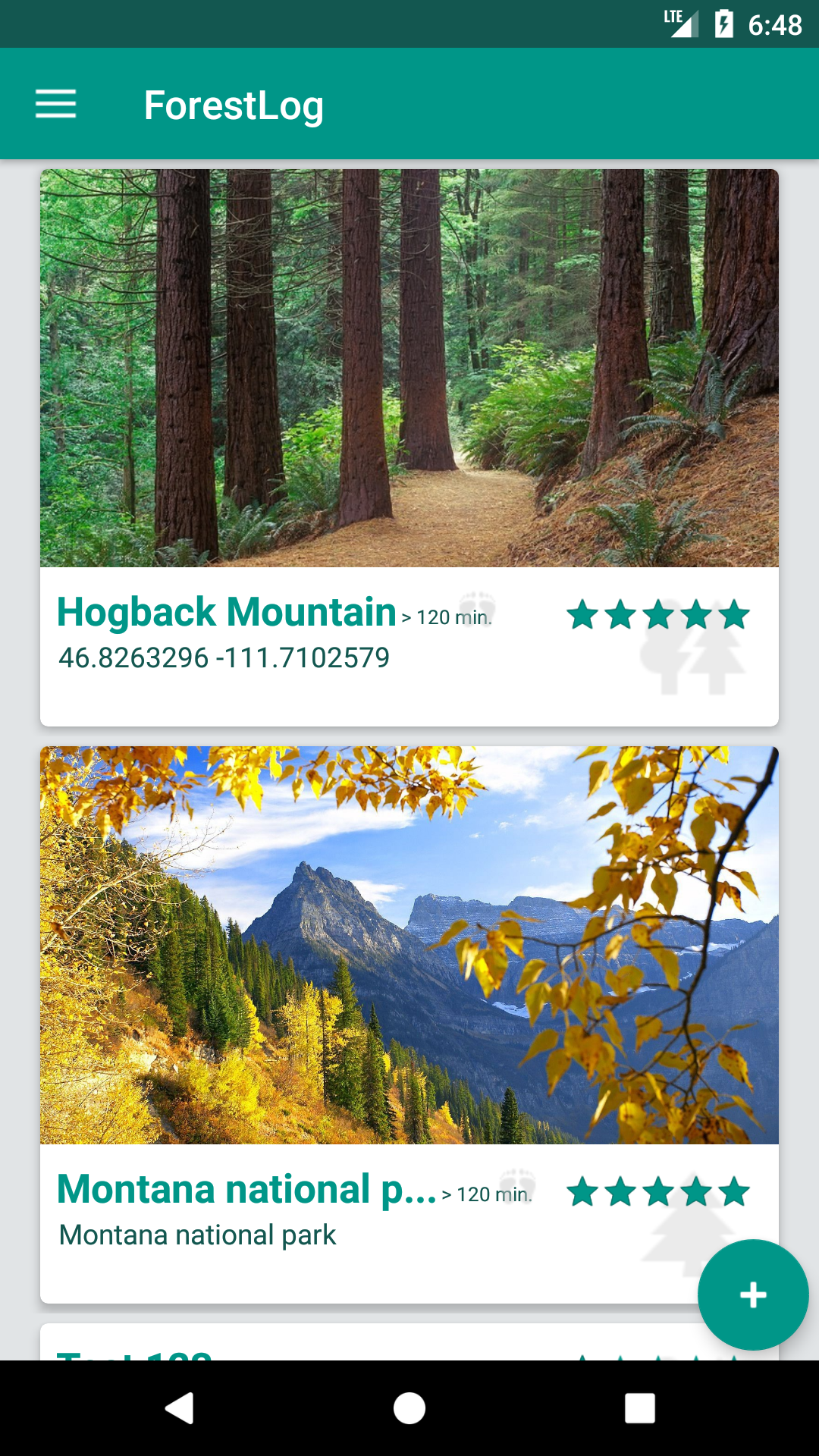This is a detailed screenshot of a mobile site. At the very top, the interface features a green header. On the far left of this header is a hamburger menu icon. Centrally positioned within the header, the text "Forest Dog" is displayed in white against the green backdrop.

Beneath this header, the main content area lists various hiking areas and trails. The first item on the list is "Hogback Mountain," which has received a perfect rating of five stars and indicates that the hike typically takes 120 minutes to complete. Following this is "Montana National Park," also boasting a five-star rating.

A prominent round button featuring a plus symbol is situated below the list, likely serving as a means to add a new hiking location to the list.

At the very bottom of the screenshot, there is a horizontal bar containing the standard navigation icons for a mobile device.